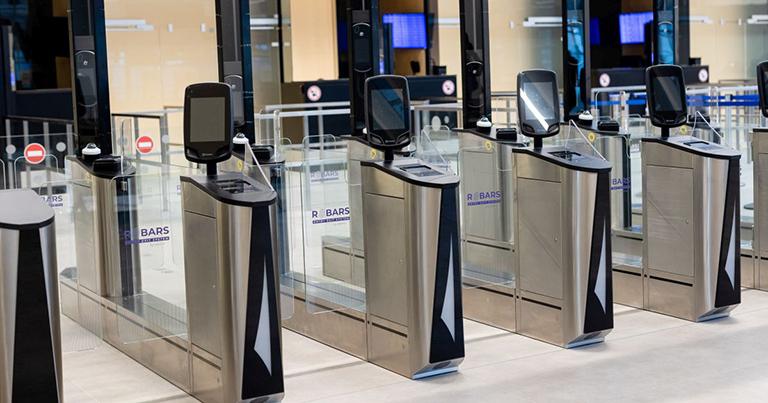The image depicts a modern, indoor security checkpoint that could be part of a subway or an airport terminal. There are six stainless steel podiums in a row, each equipped with an oblong, black-framed, digital screen. These screens, resembling oversized tablets, are mounted on metallic surfaces and are used for scanning something—possibly tickets or IDs—before passage is allowed. 

Each entrance station is defined by clear glass panels that form a barrier until the individual successfully scans their item. The glass panels feature a red circle with a white line, indicating a "do not enter" message until access is granted. The stations are separated by additional glass panes with painted bars in purple.

The setting is a spacious, well-lit room with beige walls and a clean, white-grey concrete floor. In the background, there is a flat-screen TV displaying a blue image, slightly blurred, adding to the modern and high-tech ambiance of the space. This environment suggests a controlled entry area employing advanced technology to manage the flow of people efficiently.